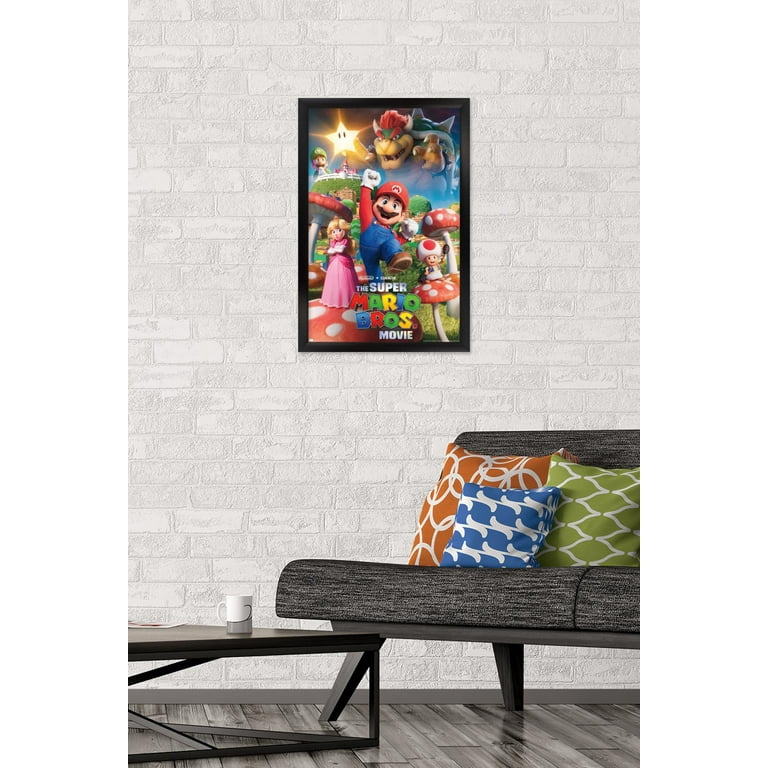This is a vertically-oriented photograph showcasing a modern living room designed to highlight a Super Mario Bros movie poster, which appears framed in black on a prominent white brick wall. At the center of the poster is Mario, accompanied by Princess Peach, Luigi, Bowser, the glowing star, and classic Super Mario mushrooms, making it a vivid and eye-catching focal point. Below the poster, a sleek, low-profile gray couch is adorned with three decorative pillows: a large orange one, a medium green one, and a small blue one, each featuring distinctive white patterns. To the left of the couch is a stylish black coffee table characterized by its intriguing leg design that interconnects in a dynamic fashion, supporting a white and gray mug. The floor is covered with grayish wood-colored tiling, enhancing the room’s modern aesthetic. The attention to detail and vibrant colors suggest this image could be part of an advertisement, whether for the poster or the living room decor itself.